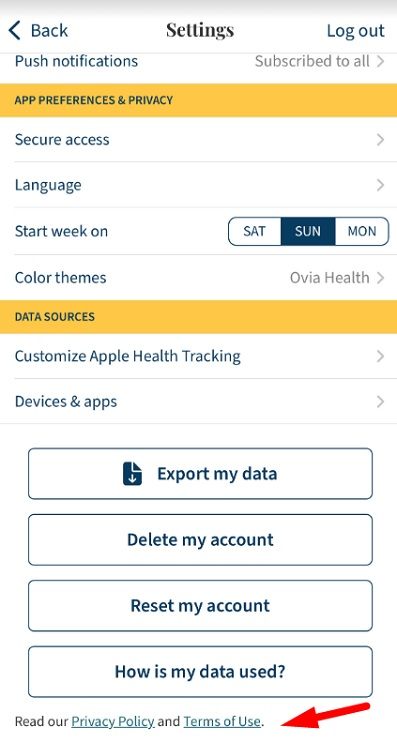The image is a long, rectangular screenshot of a settings menu, likely captured from a phone, tablet, or computer. The top section of the image displays a navigation bar with a back arrow pointing left and the word "Settings" centrally aligned. To the far right of this top bar is the option to "Logout."

Below the navigation bar is an option titled "Push Notifications" followed by an option to "Subscribe to All." The next section, titled "App Preferences and Privacy," is prominently highlighted with a light orange rectangular background and features text in a navy blue font, all in capital letters.

Following this, there is a section labeled "Secure Access," succeeded by options for "Language" settings. Further down, a section titled "Start Week On" provides three options: Saturday, Sunday, and Monday, with Sunday currently selected. The subsequent option is "Color Themes," with "OVIA Health" chosen.

The last highlighted section contains "Data Sources," also presented in navy blue font against a light orange background. This section includes options for customizing Apple Health tracking and other devices and apps, accompanied by four call-to-action buttons at the bottom.